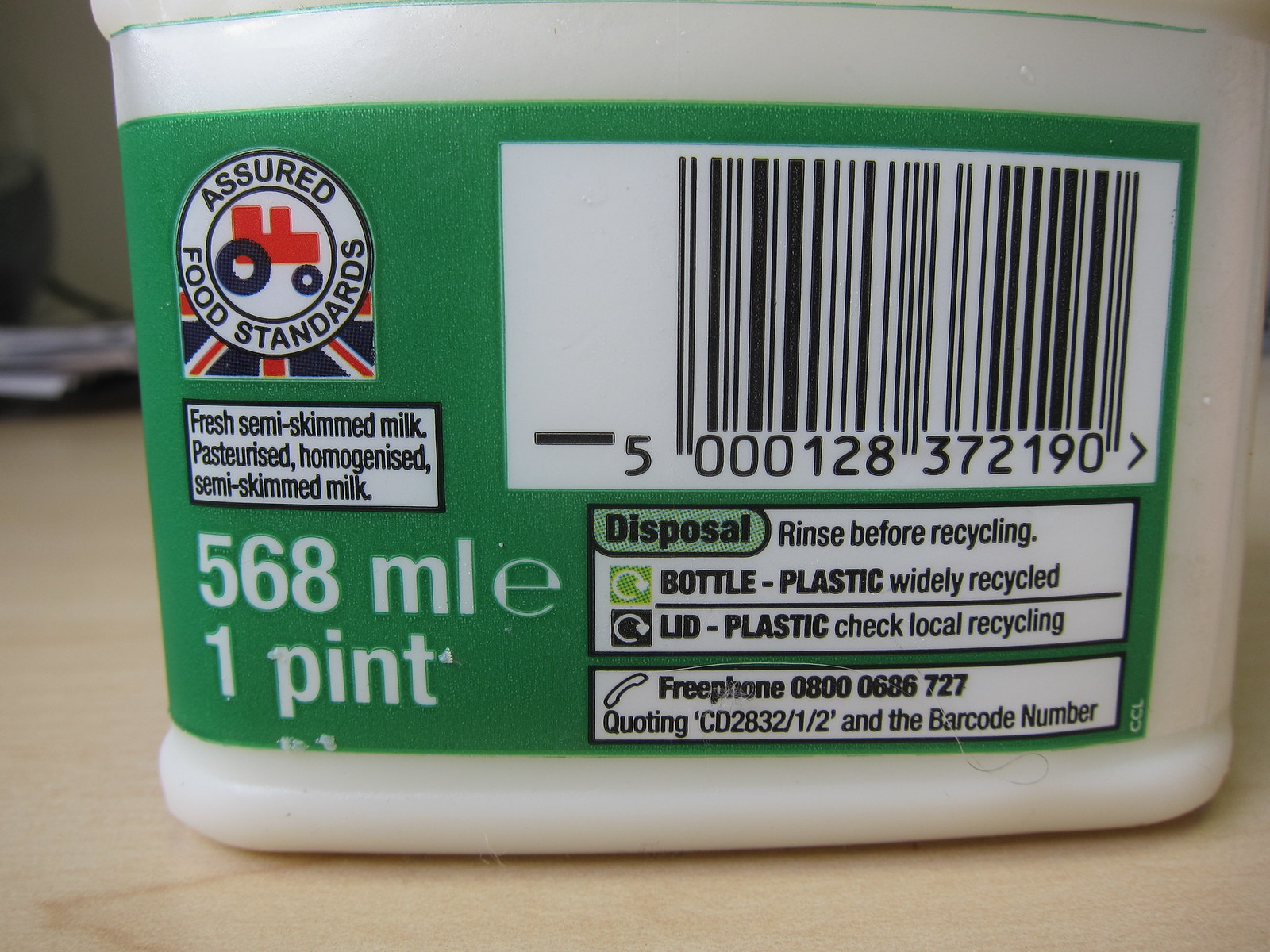The image is a close-up color photograph of the back label of a plastic white tub, which is likely placed on a brown tabletop surface with some out-of-focus objects in the left background. The label prominently features a green background with various important details. In the upper left corner, there's a circular logo with the text "Assured Food Standards" surrounding a depiction of a red tractor and a segment of the British flag. Below the logo, black text in a white box reads "Fresh Semi-Skimmed Milk," followed by "Pasteurized, Homogenized" and the measurement "568 milliliters, one pint." 

On the upper right side of the label, there's a large white box containing a barcode with the number 5000-128-372-190. Beneath the barcode, the label provides disposal instructions in a green inset: "Rinse Before Recycling," with circular arrows indicating "Bottle Plastic, Widely Recycled" and "Lid Plastic, Check Local Recycling." Further down in a black box with white text is a free phone number, 0800-0686-727, for customer queries and quoting CD 2832-1-2 along with the barcode number.